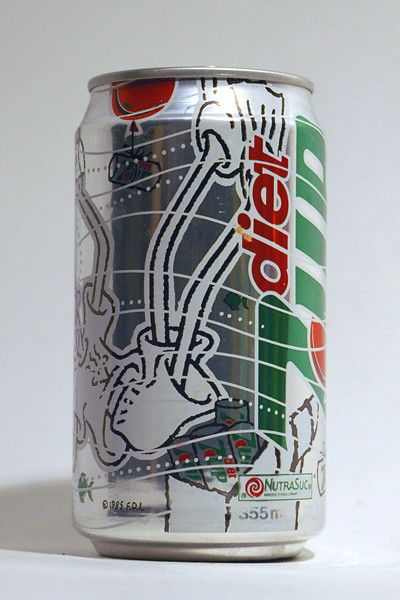This image features a tall, slender soda can of Diet 7UP, prominently occupying the majority of the frame. The label is arranged vertically with "diet" written in red lowercase letters, nestled to the left of the "7UP" logo which is aligned along the right-hand side of the can. The scene is illuminated by a light source from the right, casting a discernible shadow to the left of the can.

A whimsical cartoon adorns the can's design: a character appears to be tumbling backward with exaggeratedly skinny legs clad in flippers pointing skyward. The character sports a baggy shirt and has a pencil-thin waist complemented by spaghetti-like arms. Their left arm is raised in an upward gesture, adding to the playful motion of the illustration. A red balloon floats at the top-left of the can, echoing the same shade as the word "diet."

The branding is distinctive with its thematic colors—a monochromatic palette of black, white, and silver, seamlessly integrated with touches of red and green. The green “7UP” logo is punctuated by a red dot situated between "7" and "up." Additionally, notes on the can inform the viewer that it contains artificial sweeteners like NutraSweet or sucralose, accentuated by subtle wavy lines that add a dynamic visual texture to the overall design.